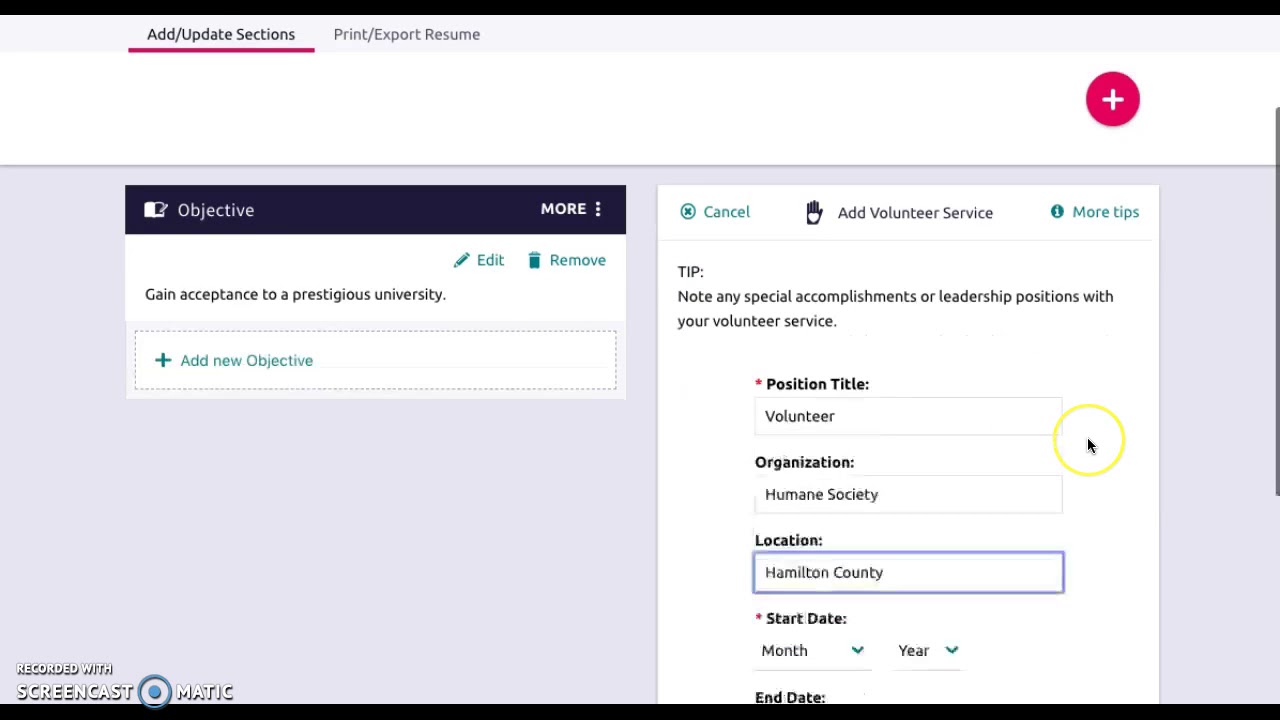This screenshot captures an interface from an application, complete with various elements and annotations. The bottom left corner features an embossed watermark in white letters with gray shadows, stating "Recorded with Screencast-O-Matic," accompanied by a blue circle with a blue dot in the center nestled between the words "Screencast" and "O-Matic." The screenshot is framed at the top by a black border and includes two menu sections in the upper left corner. One section labeled "update" has a horizontal red line underneath it, while the right section is titled "Print/Export Resume." 

In the upper right corner, there is a prominent red circle with a white plus sign. The left side of the interface features a gray background with a vertical black bar. "Objective" is displayed in white text on the left, and adjacent to it, a menu labeled "More" is indicated by three vertically aligned dots.

Beneath the "More" menu, a section on a white background includes a green pencil icon next to the word "Edit" in green lettering, followed by a green trash can icon next to the word "Remove" in green lettering. Below these options, the text "Gain acceptance to prestigious university" is shown on the left, followed by a white box intended for adding information. A green arrow labeled "Add New Objective" in green text points downward. 

On the right-hand side of the same section is a longer white area labeled "Cancel" in green. In the center, the text "Add Volunteer Service" is prominently displayed, and the far-right side features the phrase "More Tips" in green.

Three detailed text fields are located below this section, each bolded in black: "Position Title," "Volunteer Organization" (with an example entry "Humane Society"), and "Location" (such as "Hamilton County"). The fields are followed by start and end date selectors allowing users to choose the month and year. The bottom edge of the screenshot includes a black bar running horizontally across the window.